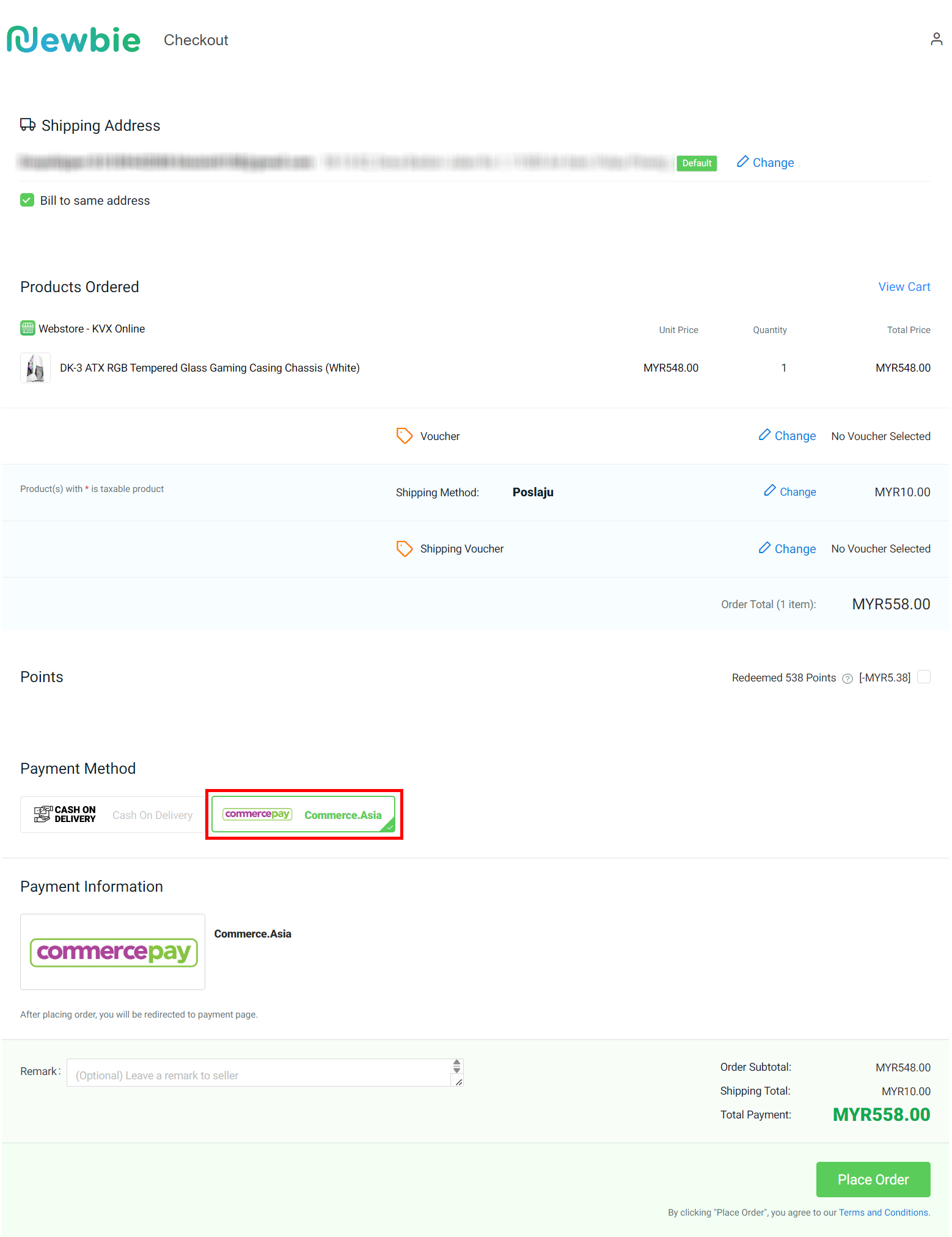This is a refined and detailed caption based on the provided information:

---

The screenshot displays a webpage from a site called "Newbie" with a distinctive logo consisting of two curved lines: a green curve at the top and a blue curve below. At the top right-hand corner, there's an icon of a truck next to the text "Shipping Address," with a blurred section below to hide private details. Adjacent to the shipping section, "Default" is highlighted in green, with an option to change it beside a pencil icon in blue.

Moving down, a green checkmark indicates that the billing address is the same as the shipping address. Further below, the section "Products Ordered" is displayed in black text. A green box appears below with the label "Web Store - KVX Online." On the far right, "Cart" is highlighted in blue. Directly under the web store information is an image of the ordered product, which is a "Tempered Glass Gaming Glass White" listed with a unit price of $5.48, quantity of one, bringing the total price to $5.48. 

A blue box notes that the product is taxable, marked with a red asterisk, and incurs a $10 shipping fee via POS Laju. An option to apply vouchers and change the shipping method is provided. The order total is noted as MYR 558.00, with the user earning points for their purchase—538 points mentioned after deductions. Payment methods available include Cash on Delivery and Commerce Pay, with the latter being selected. 

At the bottom, a green "Place Order" button is present, summarizing the total payment amount.

---

This caption accurately conveys the contents of the screenshot in a clear and organized manner.